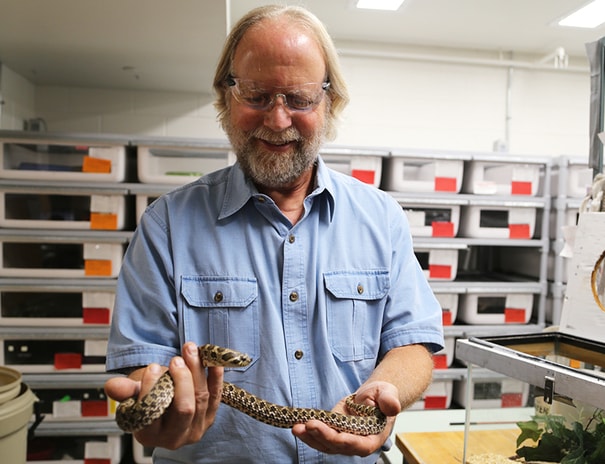The image captures a color photograph of a man, likely a herpetologist or reptile collector, standing in a well-lit room with drop ceilings and large troffer fluorescent lights, suggesting he may be in an academic building or possibly a private residence. The room is lined with sturdy, gray, plastic storage shelves filled with labeled bins, presumably containing snakes. The man is in his 50s or 60s, with a receding hairline but long gray-blond hair, wearing safety goggles and a light blue, short-sleeved denim shirt with two pockets. He sports a salt-and-pepper mustache and beard. Smiling down at the snake he's holding, he has the reptile's head carefully clamped between his fingers. The snake, notable for its beautiful net-like pattern, might be a rattlesnake or a hognose. Beside the man is a glass terrarium with a wooden frame and mesh top, containing plants. A garbage can is visible at the lower right corner of the image.